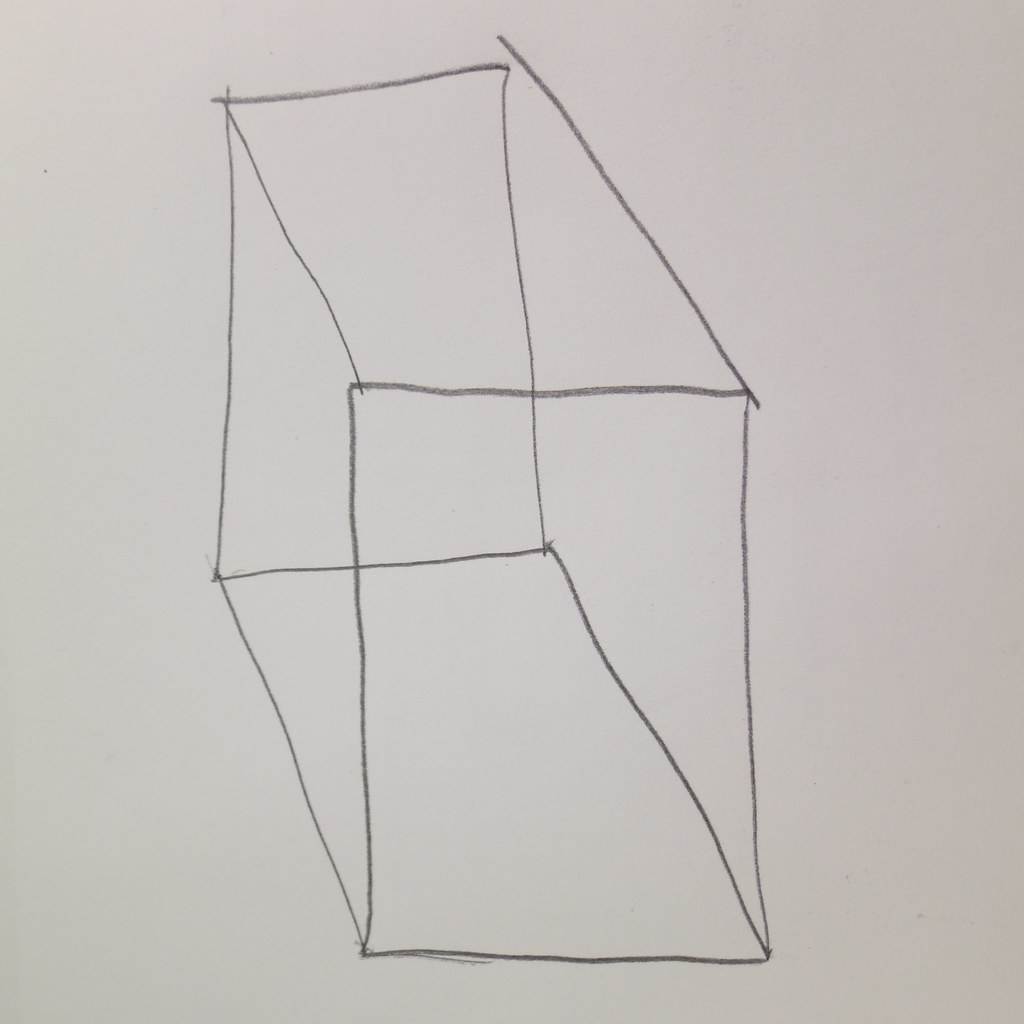The image captures a photograph of a hand-drawn sketch made on a standard white sheet of printer paper. The drawing, done in gray pencil, appears to depict a three-dimensional cube or a rectangular prism with elongated lines suggesting depth. The artist attempted to illustrate the geometric shape by including an angled rectangle for the top face, with corresponding lines extending downwards to form the sides. The bottom panel is also visible, connecting to the right side panel of the shape. However, the lines are not meticulously aligned; in particular, the upper right corner shows a line extending off without meeting the adjacent edges, resulting in an incomplete connection. Additionally, other points of intersection exhibit overlapping lines, indicating a casual and imprecise approach to the sketch.